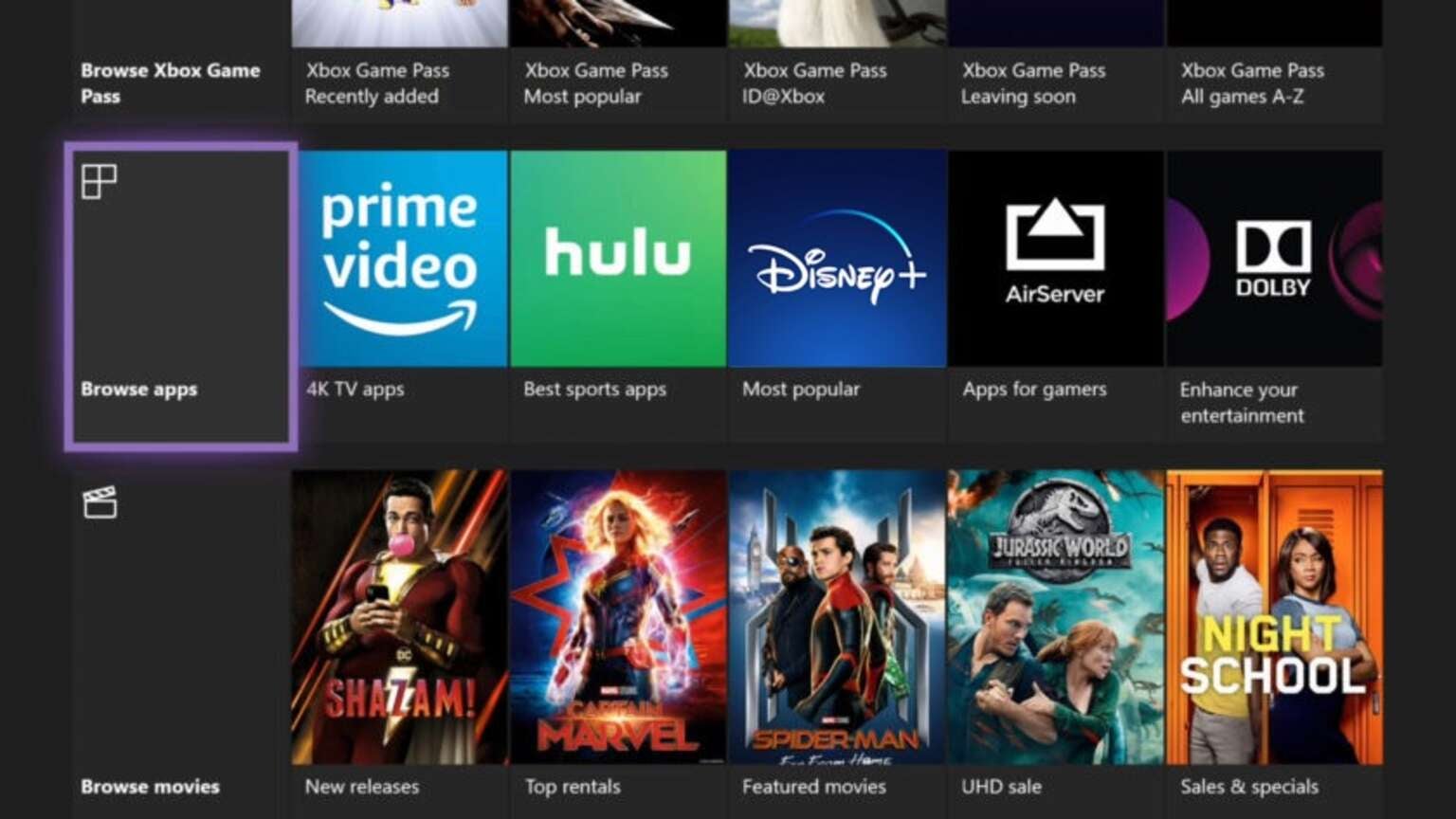This appears to be a screenshot of a browsing page for Xbox content, displaying various games, apps, and movies. The page is structured with a grid of rectangular items, organized into different sections. On the left sidebar, there are three main categories: "Browse Xbox Game Pass," "Browse Apps," and "Browse Movies."

Within the "Browse Xbox Game Pass" section, there are five subcategories listed:
1. **Recently Added**
2. **Most Popular**
3. **ID Added**
4. **Leaving Soon**
5. **All Games A-Z**

Each subcategory showcases a selection of games available for the Xbox Game Pass.

In the "Browse Apps" section, five highlighted applications are shown:
1. **Prime Video** - Streaming service with diverse content.
2. **Hulu** - Another streaming service offering TV shows and movies.
3. **Disney+** - Platform for Disney’s vast library of films and series.
4. **AirServer** - App for screen mirroring and streaming.
5. **Dolby** - App focused on enhancing audio-visual experiences.

Each app has a brief description beneath it.

Finally, the "Browse Movies" section features five popular films:
1. **Shazam!** - A superhero movie with a lighthearted tone.
2. **Captain Marvel** - A Marvel Cinematic Universe film featuring the titular superhero.
3. **Spider-Man** - Likely a film from the various Spider-Man franchises.
4. **Jurassic World** - A movie from the Jurassic Park series, centered on a dinosaur theme park.
5. **Night School** - A comedy film about adults attending night school.

This detailed layout helps users easily navigate and choose from the various entertainment options available on Xbox.